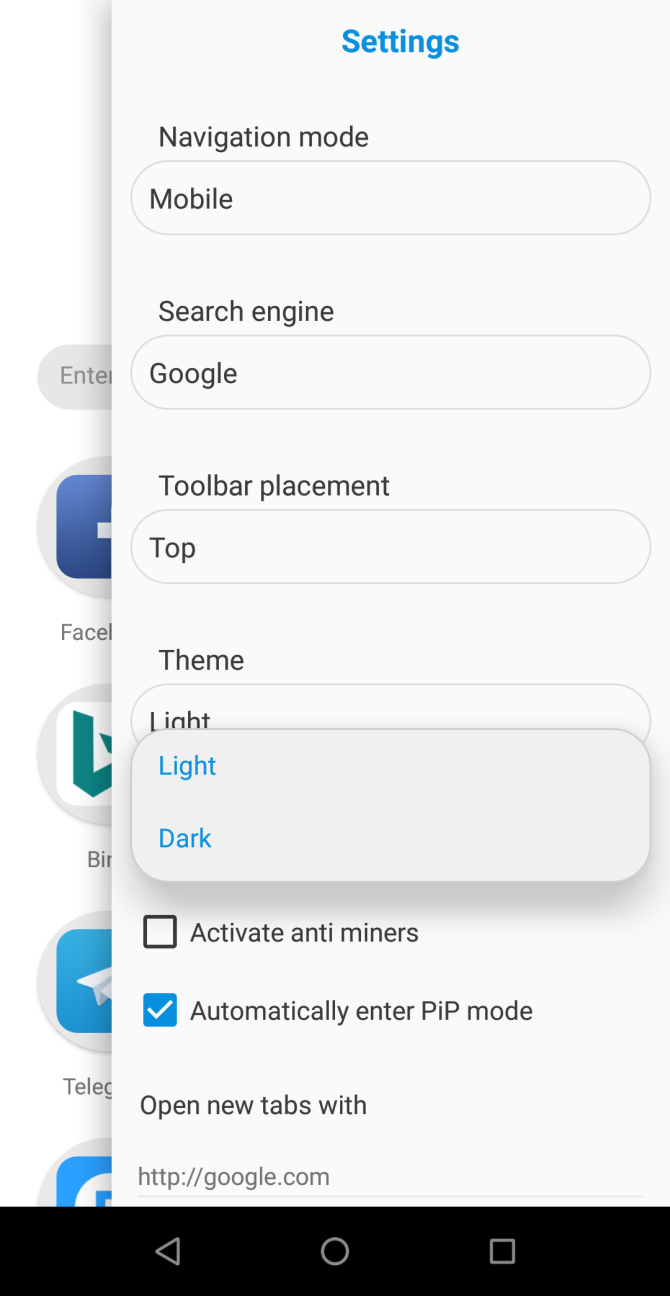This image is a screenshot of a smartphone displaying a settings page in portrait orientation, with proportions typical of a mobile device. The central feature of the image is a prominent pop-up settings window occupying around 70% of the screen's width from right to left. This settings window has a blue header labeled "Settings," a gray background, and contains multiple option sections with selectable items.

The first section, titled "Navigation Mode," includes an option labeled "Mobile" encased in an oval. Below it, the "Search Engine" section lists "Google." The "Toolbar Placement" option is set to "Top." The "Theme" section offers "Light" and "Dark" modes, with "Light" currently selected, though both options are highlighted in blue.

Additional settings include a checkmark beside "Activate Anti-Miners," indicating the option is enabled. Another checked box is labeled "Automatically enter PIP mode." There is also an option to "Open new tabs with google.com."

In the background of the image, several mobile app icons are partially visible, including Facebook, an app starting with "BIR," Telegraph, and possibly other applications. At the bottom of the screen, a navigation bar features a left-pointing triangle, a circle, and a star icon. This bar likely represents the phone's navigation controls. Overall, the image captures the customization of various default settings on a smartphone.